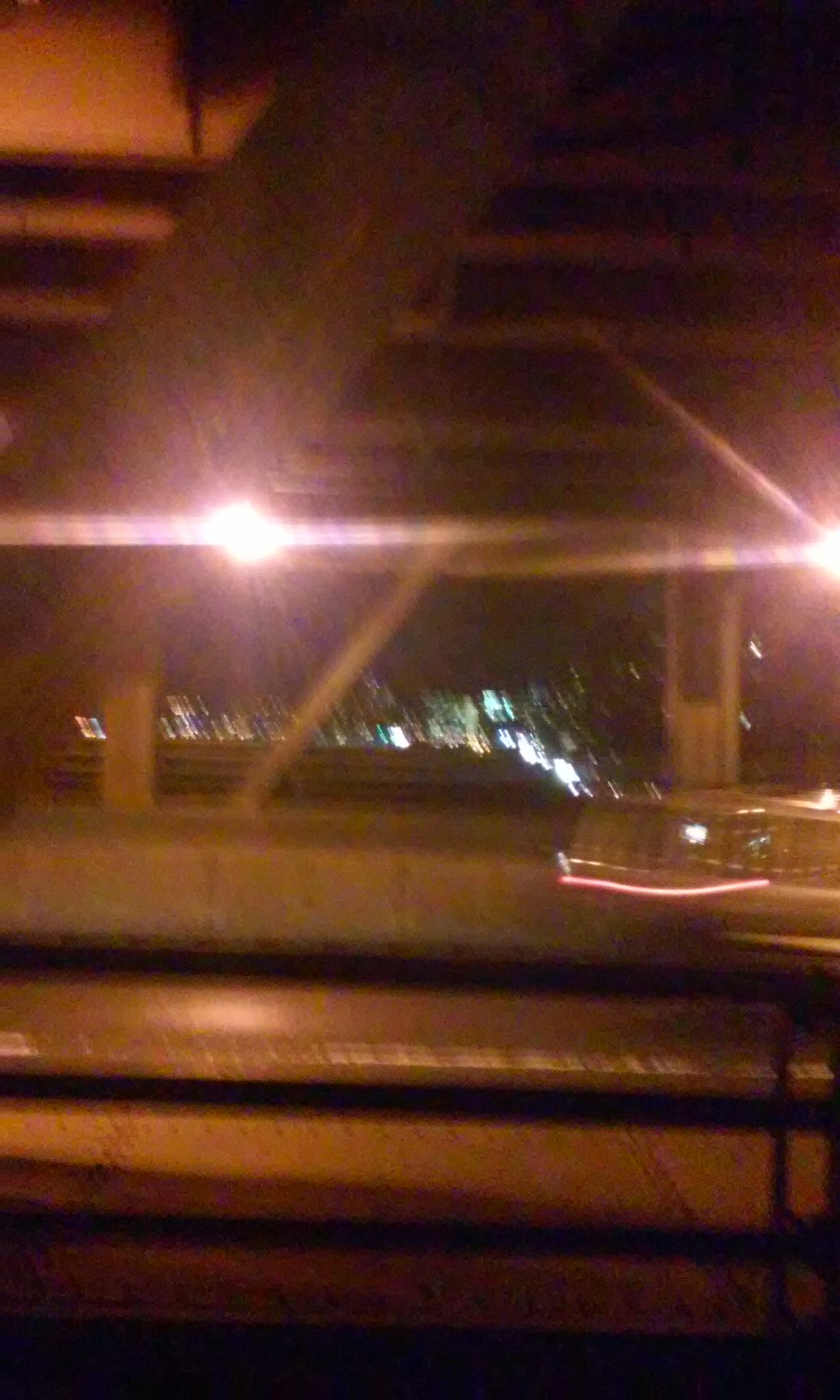The image depicts a blurry, nighttime view taken from inside a moving car, likely while driving under the underside of a large, concrete bridge or overpass. The poor quality of the photo, with its fuzzy appearance and obstructive, circular bright lights shining directly toward the camera, contributes to the difficulty in discerning details. However, visible are concrete pylons at the corners of the bridge support structure and an overhead stretch of what appears to be large steel girders. A median runs beneath the bridge, and a fence separates the road from the camera's vantage point. In the distance, city lights illuminate the horizon, possibly from buildings, with silhouettes of trees faintly visible. Overall, the chaotic composition and movement hint at the spontaneous nature of the photo.